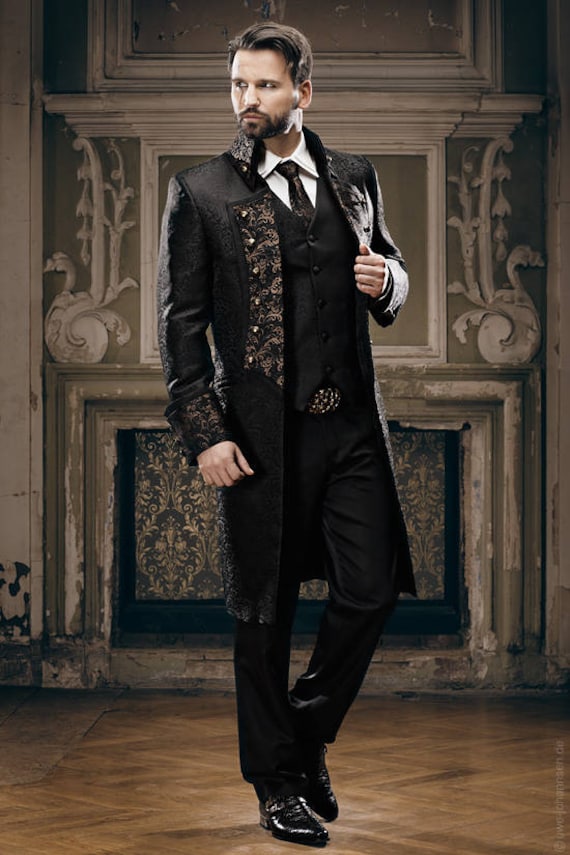This is a portrait-style photograph in a tall, rectangular format, featuring a young white man, possibly in his 20s or early 30s, as the central figure. The man is standing on a brown tile floor in front of a detailed, vintage-style background. The background showcases an ornate, Rococo-style carved fireplace with green floral wallpaper seen through the empty fireplace. The fireplace itself has a chipped wood mantle in white and green, embellished with intricate carvings.

The man has light skin, dark ear-length hair combed to the side, and sports a well-groomed beard and mustache. He is dressed in a striking, colonial-era-style outfit: a long, knee-length black coat adorned with goldish floral designs on the sides and collar. Beneath the coat, he wears a white dress shirt with a tie, a vest, a metal belt, brown pants, and shiny black dress shoes. His body is slightly tilted to the right, while his head is turned to the left, looking away from the center of the frame.